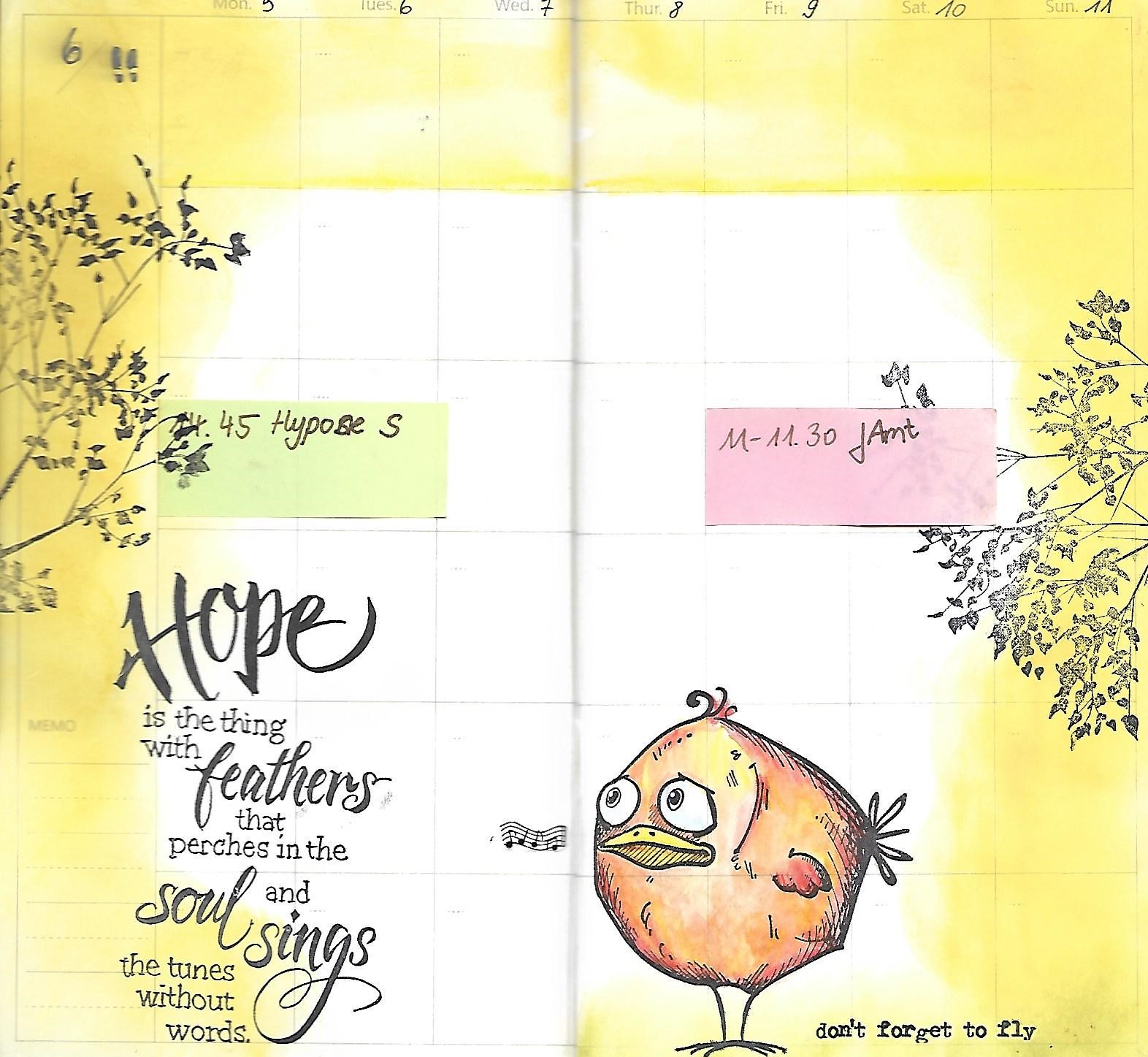The image depicts a calendar planner with a predominantly yellow hue, accented by illustrated branches and leaves along its edges. The calendar design features a white center and displays the days of the week at the top. On the left-hand side, there's a green post-it note with the text "445 Hypos S." A pink post-it note on the right side reads "M1130JAMT." In the bottom left quadrant of the calendar, a quote reads, "Hope is the thing with feathers that perches in the soul and sings the tunes without words." The bottom right quadrant showcases a hand-drawn, chubby, and slightly fearful-looking bird standing on its legs, accompanied by the words, "Don't forget to fly."